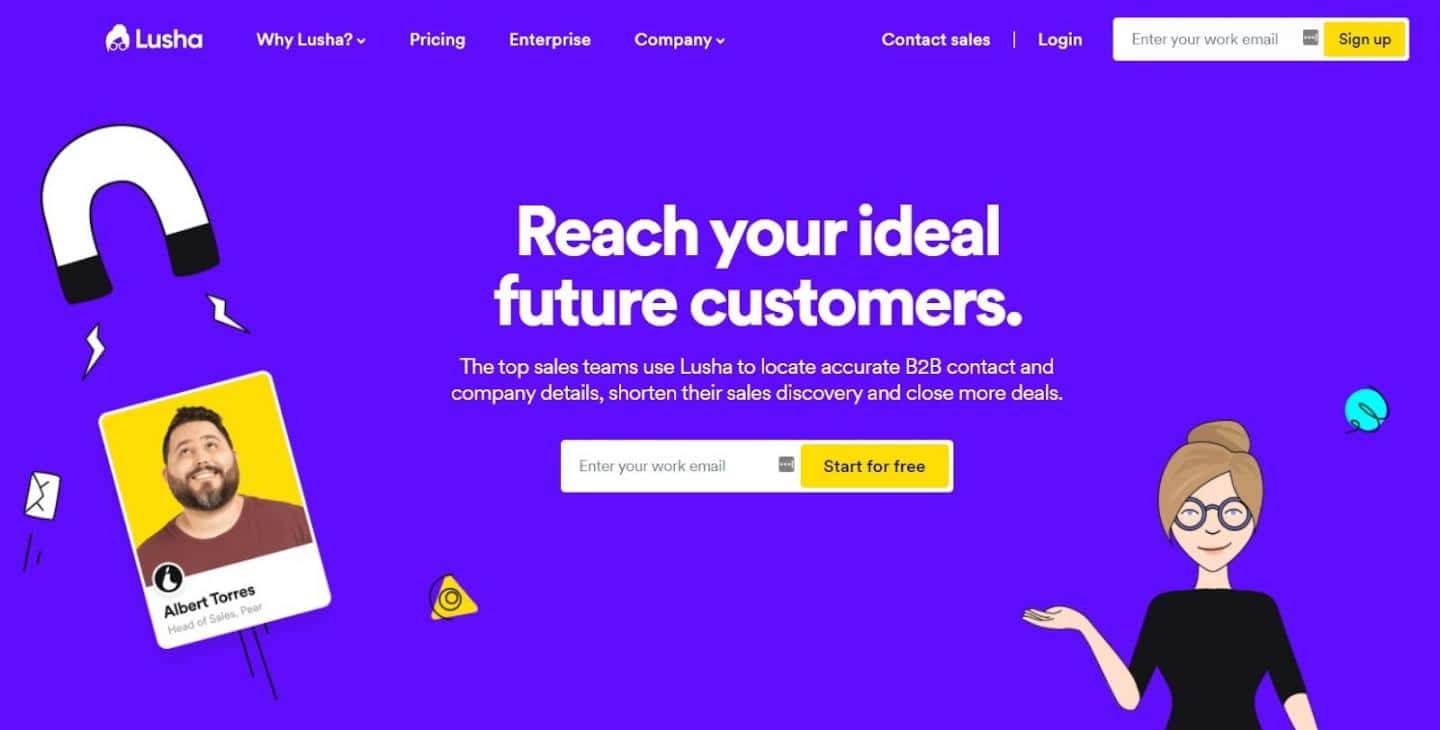The website homepage for Lusha features a vibrant purple background that immediately catches the eye. In the upper left corner, the Lusha logo is prominently displayed. This logo, a unique design, resembles a tall, white wig paired with a set of glasses or sunglasses, though no face is depicted.

At the top of the page, there is a navigation bar with several menu options: "Why Lusha" (which expands to a drop-down menu), "Pricing," "Enterprise," and "Company" (another drop-down menu). To the far right, you’ll find links for "Contact Sales" and "Login." In the very top-right corner, a search box is situated beside a yellow button labeled "Sign Up," where users are prompted to enter their email address to begin the registration process.

Dominating the middle section of the webpage is bold, white text that reads, "Reach Your Ideal Future Customers." This is followed by a subheading that explains, "Top sales teams use Lusha to locate accurate B2B contact and company details, shorten their sales discovery, and close more deals." Beneath this text, there is an email entry field along with a yellow button that invites users to "Start For Free."

To the left of this sign-up section, there is a visually engaging illustration: a cartoon-style magnet in white and black. This magnet appears to attract a cartoonish image of a man—named Albert Torres—who looks up at it with interest. In the lower right part of the screen, another cartoon figure, a woman, is depicted. She wears a black shirt and black-rimmed glasses, and her hair is styled in a beehive fashion, reminiscent of a honeybee’s look.

The cohesive design and illustrative elements on the Lusha website create an inviting and user-friendly interface, designed to attract and engage sales professionals.